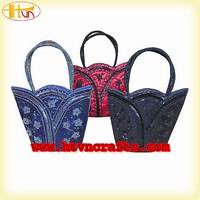The advertisement shows three handbags positioned in a triangular fashion on a white background bordered by a yellow frame. The frontmost handbag to the left is blue with a light blue floral pattern. The frontmost handbag to the right is solid black, and it is unclear if it has any patterns due to the grainy quality of the image. The handbag at the back, forming the top of the triangle, is red with a fancy black design that includes patterned triangles. A URL, though too small and blurry to decipher fully, is printed in red at the bottom of the image, likely containing "www" and "Nora." In the top left corner, there is a logo that appears to combine a sideways "S" with possibly a trumpet or the letters "H" and "S" in yellow and red.